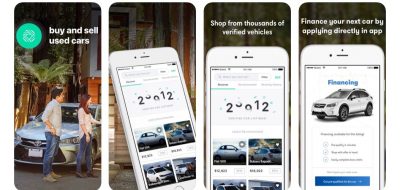This image features a series of four side-by-side screens, each resembling a cell phone display:

1. The first screen depicts a man and a woman standing beside a silver-white car. The scene is set against a generic outdoors background, suggesting a driveway or dealership lot. At the top, bold text reads "Buy and Sell Used Cars," indicating a platform for trading pre-owned vehicles.

2. In the second screen, a close-up of a cell phone is shown, displaying a car-buying website. This screen's backdrop includes a construction site with a partially built wooden house, subtly indicating that car buying can be done on-the-go or from any location.

3. The third screen presents another cell phone held upright, displaying the phrase "Shop From Thousands of Verified Vehicles." The background is a decorative, floral-patterned wallpaper, adding a touch of elegance and comfort to the user experience.

Overall, the images collectively convey a seamless and versatile car-buying experience facilitated through mobile technology.